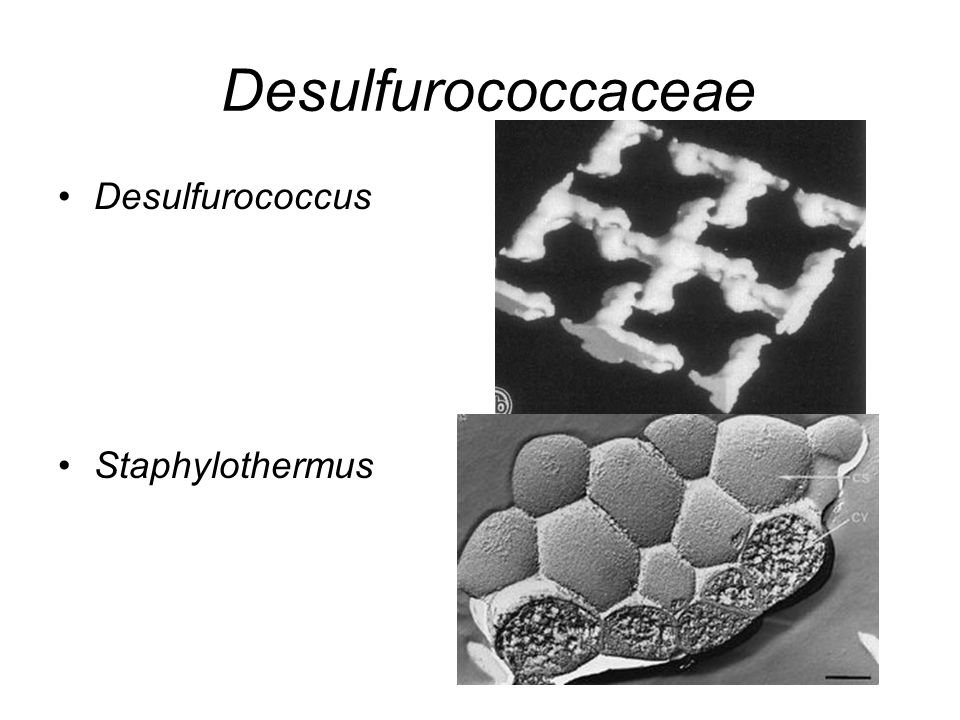The image is a black and white slide from what appears to be an educational PowerPoint presentation or textbook page about two types of biological compounds or bacteria. The slide, which has a white background, is titled "Desulfurococcaceae" in black text at the top. Below the title, there are two bullet points. The first bullet point reads "Desulfurococcus," accompanied by an image on the right that depicts objects with a squiggly-line pattern forming a box with a cross inside, which subdivides into four squares. The second bullet point reads "Staphylothermus," next to an image resembling a turtle shell made up of nine circular plates and a textured grouping at the bottom, which looks like five pouches of dirt in various shades of gray.